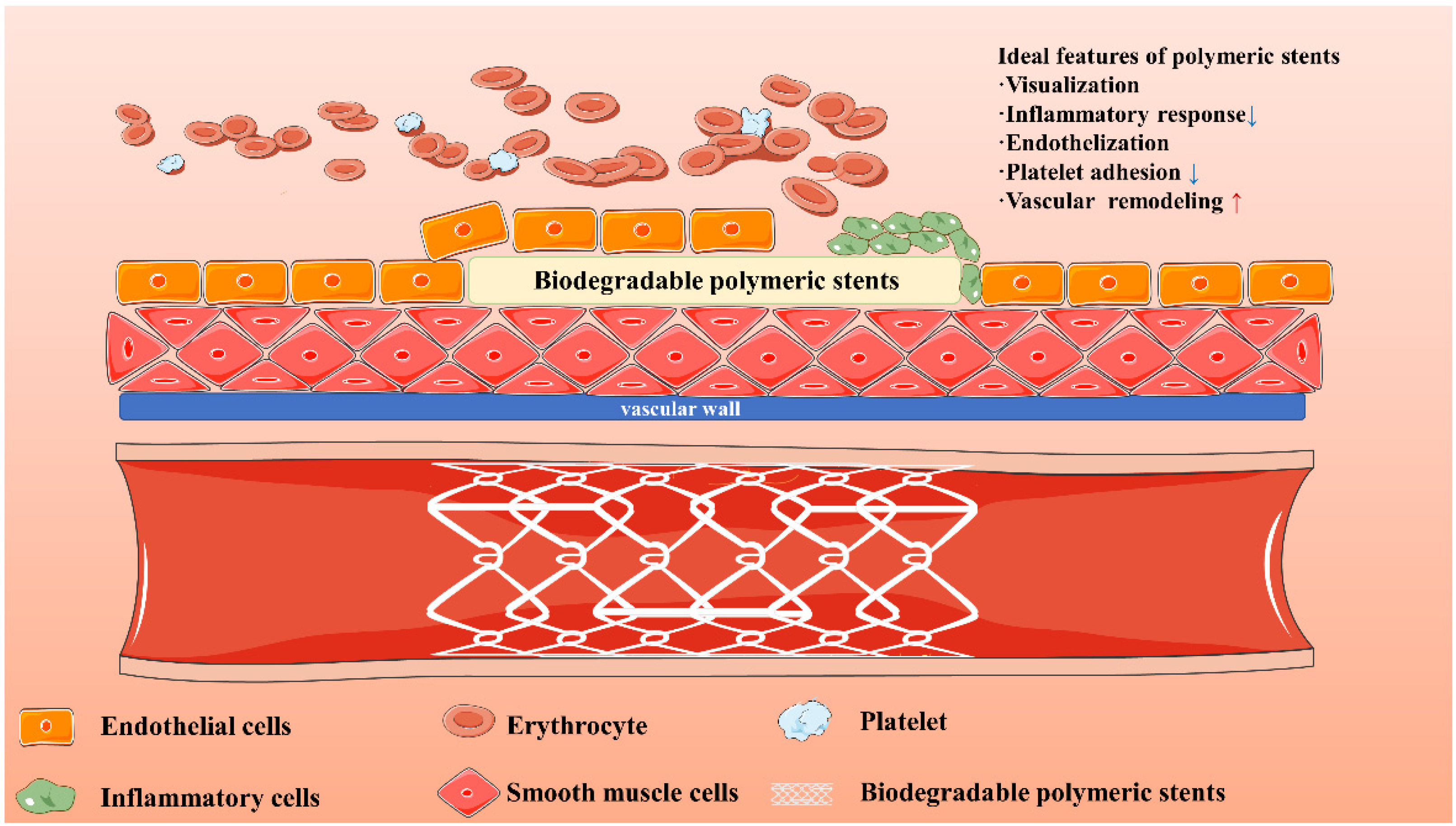The image appears to be an illustration from a medical textbook or an informational pamphlet about biodegradable polymeric stents, likely used in cardiac procedures. The central visual is a cross-section of an artery, where various stents are depicted in a row, though four stents are shown out of place with green elements indicating some process or component. The vascular wall, highlighted in blue, alongside a red-painted depiction of the artery's interior, features white designs symbolizing platelets. The illustration is labeled with key features and ideal characteristics of these stents, including visualization, inflammatory response, endothelialization, platelet adhesion, and vascular remodeling. Additionally, different cell types such as inflammatory cells, endothelial cells, erythrocytes, and smooth muscle cells are identified, providing a comprehensive overview of how these stents function and interact within the vascular system.